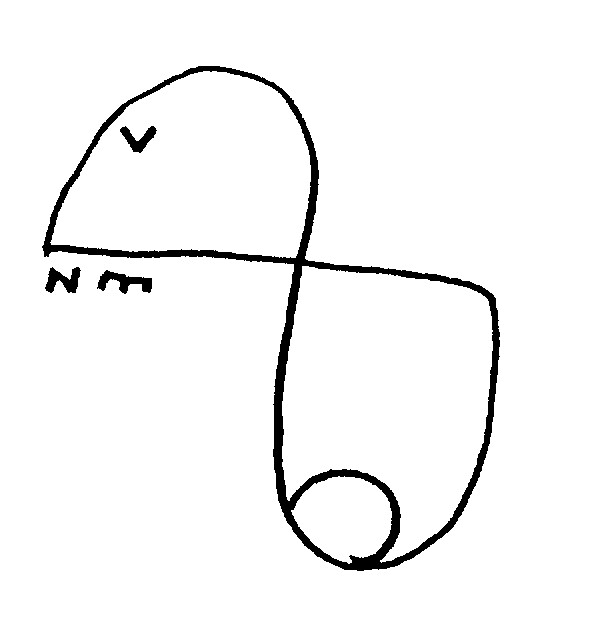This image features an extremely minimalist line drawing, evocative of a bird. The composition consists of a single, continuous line that traverses from left to right across the center of the canvas, creating a foundational horizontal axis. From the left endpoint of this line, an upside-down U extends upward, forming the bird's head-like structure, with its apex reaching the midway point of the horizontal line. Below this central line, a larger, inverted U sweeps downward, suggesting the body of the bird, connecting the midpoint of the line to its right endpoint.

Within the upper U, a small V-shaped indentation serves as a simplistic representation of eyes, inviting the viewer to employ a bit of imagination. Beneath the horizontal line, nestled between its midpoint and the bottom of the larger U, an abstract N and M configuration hints subtly at a beak or perhaps teeth-like elements, adding a touch of enigmatic character to the figure. At the very bottom of this lower U, a crescent moon shape is integrated, simulating a tail and completing the portrayal with a hint of whimsy. The overall design is a compelling exercise in minimalism, leaving much to the viewer's interpretation while suggesting the essence of a bird.